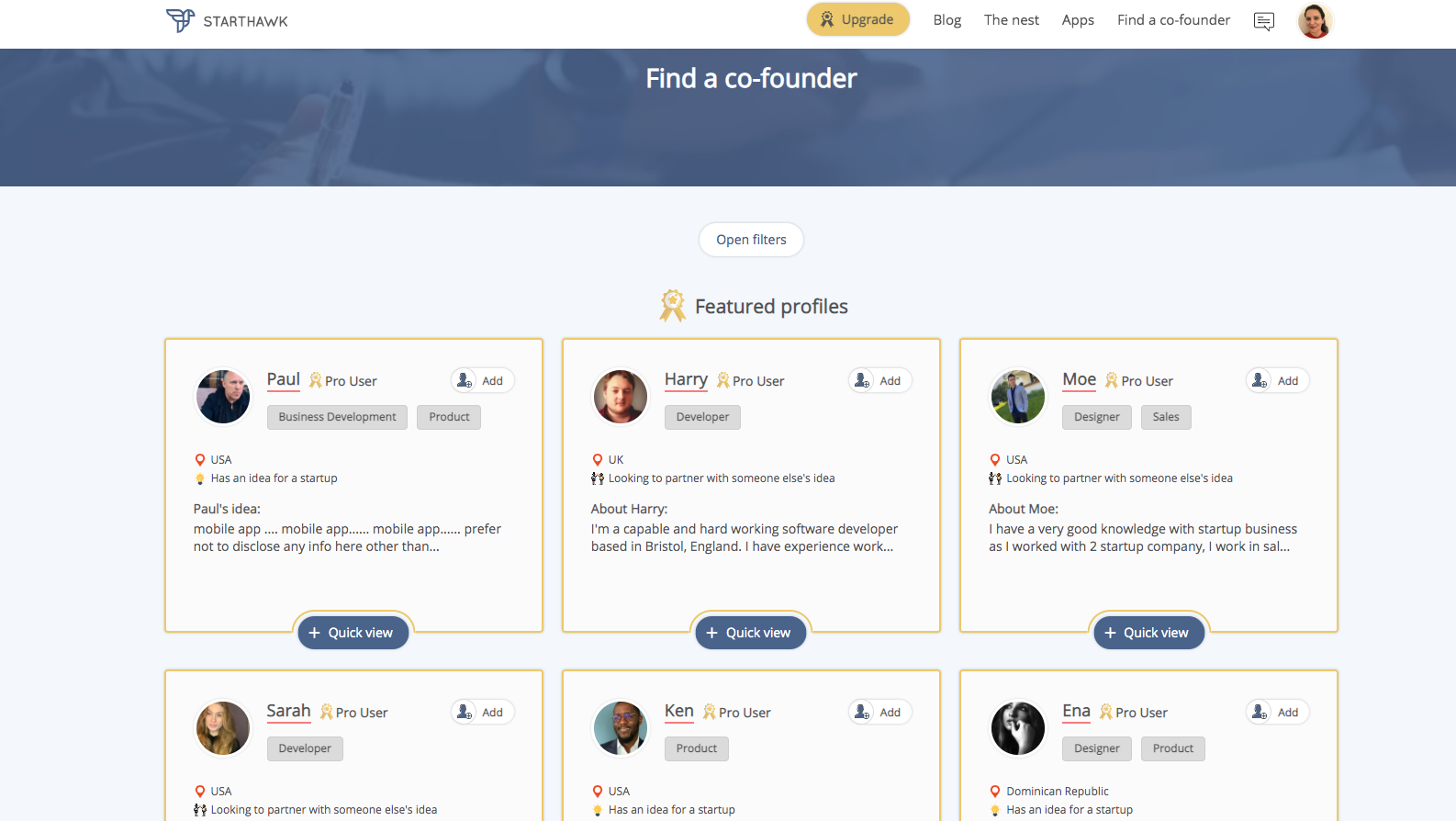The image features a long rectangular banner with a blue background. Prominently displayed in the center is the text "Find a Co-founder." In the upper left corner is the logo "starTHAWK." To the right of the logo, there is a small circular image of a girl with long, dark hair.

Below this, the banner introduces various profiles. First is Paul, depicted as an older man wearing a black shirt. Paul is a pro user from the USA with ideas for a mobile app, although specific details are not disclosed.

Next is Harry, who appears to be in his early 40s. Harry is a capable and hardworking software engineer based in Bristol, England.

Following Harry is Moe, who has extensive knowledge of startup businesses.

Underneath Moe's profile is Sarah. Her name is underlined in red, and she has shoulder-length blonde hair. Sarah is wearing a black shirt and is based in the USA.

Ken is the next profile listed. His name is also underlined in red. Ken is a pro user wearing glasses and a suit jacket. He is based in the USA and has an idea for a startup.

Finally, there is Ena from the Dominican Republic, who has long dark hair.